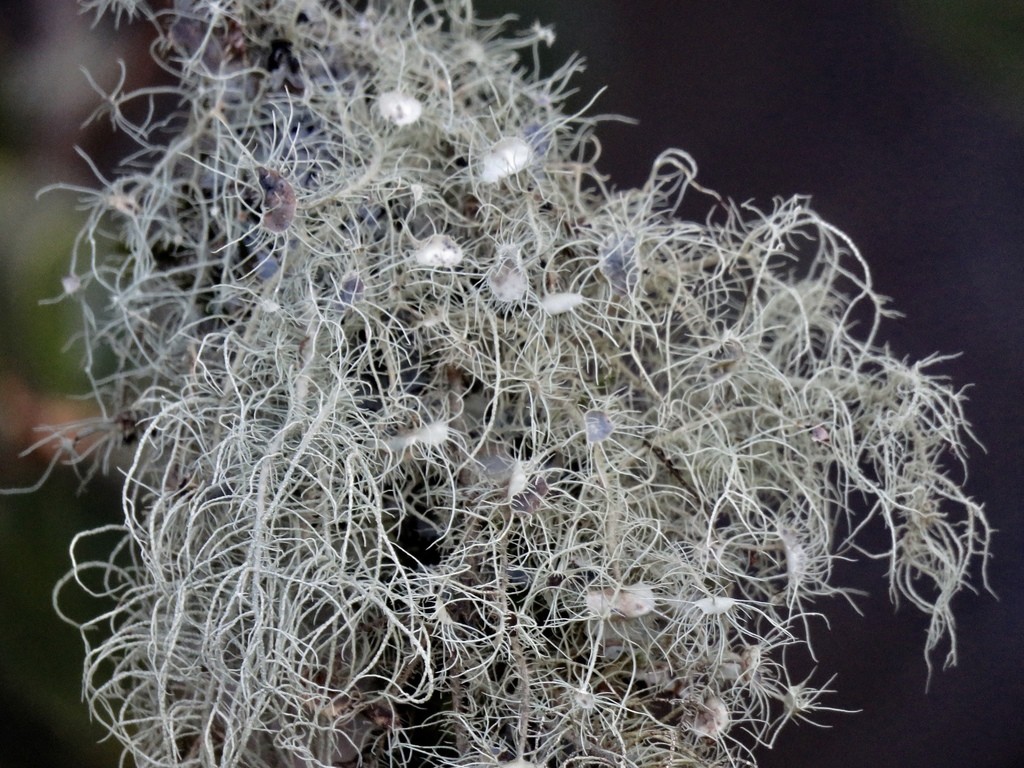The image is a macro, photographic close-up of a botanical structure, possibly Spanish moss or a similar plant. The setting appears to be outdoors. The scene is dominated by a mass of wiry, white branches that occupy most of the frame. Interspersed among the branches are approximately six or seven small, oval-shaped white blobs, which resemble animal heads, some featuring what looks like eyes. These branches and blobs create a wispy, fur-like appearance. 

The top left corner highlights a gray glob with white spiny projections, contrasted against a blurred background. The background itself is a gradient of out-of-focus colors; with the top left corner displaying hints of green and pink, transitioning to medium blue on the right side, and incorporating shades of gray, beige, and light brown. No text is present in the image. The overall composition, featuring dense and less dense clusters of these white fibers, suggests a dendritic, almost mop-like quality.